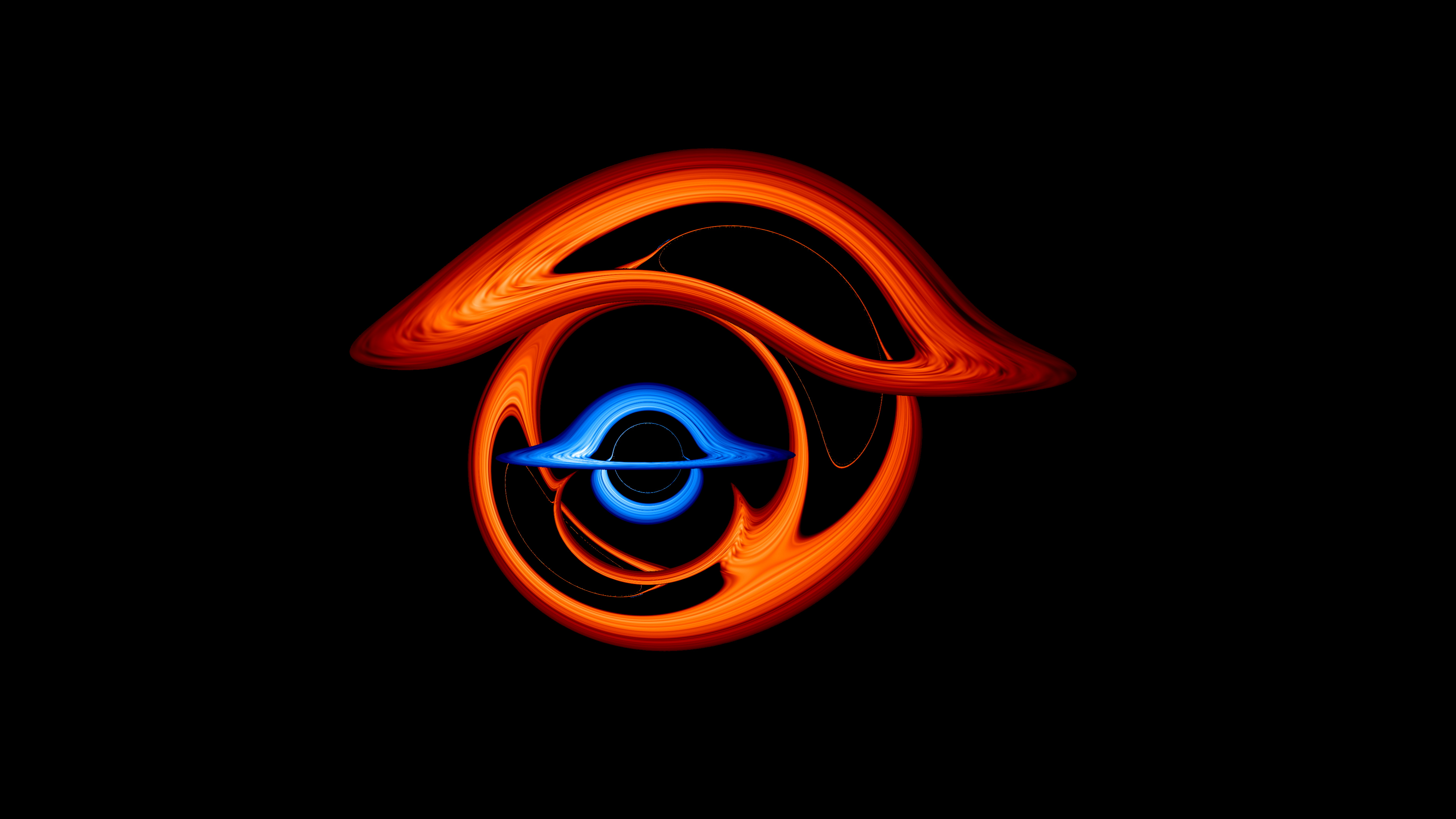The image in question is an abstract, artistic creation set against a pitch-black background. Dominating the center, vibrant swirls of reddish-orange and bright blue create a dramatic, eye-catching spectacle. The red-orange elements appear like molten lava or wavy, stretching plastic, possibly evoking the feeling of energy swirling around a black hole. This dynamic, fiery swirl seems to wrap around a smaller, yet equally vibrant blue nucleus that resembles a planet or a concentrated form of energy, slightly oriented to the left of the center. The overall composition presents a striking, almost cosmic aesthetic, with the vivid colors and flowing shapes converging into an eye-like focal point, making it a compelling visual feast that could be recreated in neon.